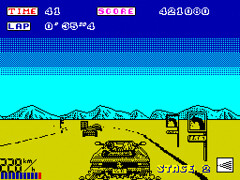The image appears to be a screenshot from a retro-style car racing video game set in a desert environment. The car, which is moderately centered on the screen, is speeding along a yellow desert landscape with a vividly blue sky overhead. In the background, there are rugged mountains that add to the desolate yet picturesque scenery. A small white lake can also be seen, contrasting sharply with the yellow sands. 

Situated at the top of the screen is the game interface, which includes a timer whose numbers are not clearly visible, along with a lap counter displaying "Lap: 0/35/4." The player's score is prominently shown as "421,080." At the bottom left corner, the car’s speed is indicated as "220 km/h." Just to the right of the car, there is an indicator that reads "Stage 2," suggesting the progression level within the game. Additionally, a couple of colorful banners can be observed flanking the track, and there are a few other cars ahead of the player's vehicle, adding to the competitive atmosphere.